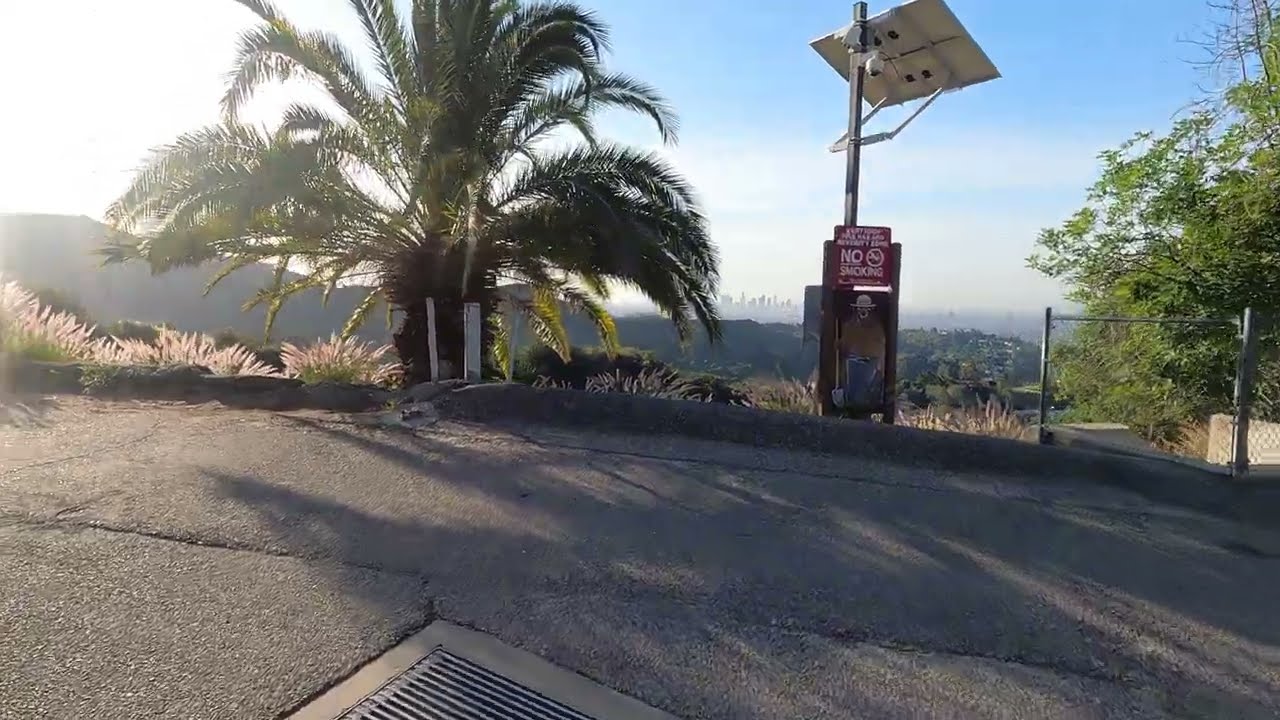The image depicts a city overlook taken on a sunny day. The scene is anchored by a cracked asphalt road with a metal grate in the lower left half. To the right, a slightly bent chain-link fence runs alongside a drainage ditch filled with trees. Dominating the upper center is a short palm tree with lush green leaves. Adjacent to the palm tree stands a light post adorned with a red "No Smoking" sign featuring white text and a crossed-out cigarette icon. Below this sign is a painting of a man in a brown shirt and blue jeans, holding a wood-handled, metal-headed shovel. The sky above is a brilliant blue, layered with white clouds, and the upper left corner is particularly bright, likely due to direct sunlight. In the distant background, the outline of hills or mountains is faintly visible, adding depth to the landscape. There are no buildings, cars, or people in sight, contributing to the serene atmosphere highlighted by sun rays permeating the scene.